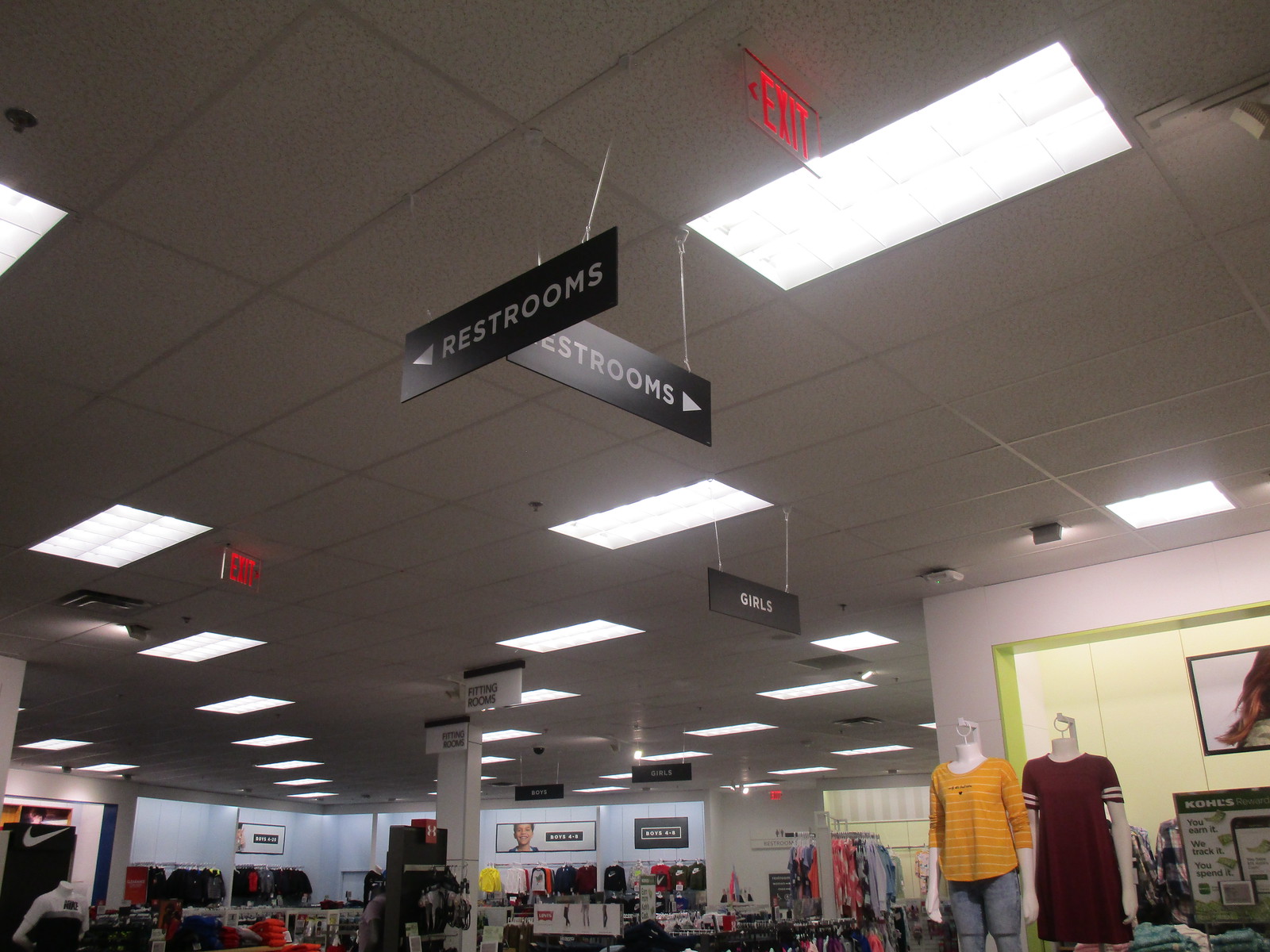This angled photograph captures an indoor view of a department store, taken slightly upward toward the ceiling. The ceiling is adorned with white, rectangular tiles and is well-lit by several bright white light fixtures. Prominent in the scene are several clothing racks populated with various garments, indicating an extensive shopping area.

Hanging from the ceiling are black signs with white font, giving directions: restrooms can be found to both the left and straight ahead, while the area being viewed primarily caters to the girls' clothing section. Additionally, a white sign directs customers to nearby fitting rooms.

In the lower right corner, there are two mannequins on display. One mannequin, complete with a head, is dressed in a yellow long-sleeve shirt and blue jeans, presenting a casual outfit choice. Right beside it, a headless mannequin sports a purple-brown short-sleeve t-shirt, offering another apparel option for customers.

The store's interior walls are white, though there are hints of greenish hues in the background, suggesting the vicinity of the fitting rooms. This detailed composition offers a clear and organized shopping environment for store visitors.